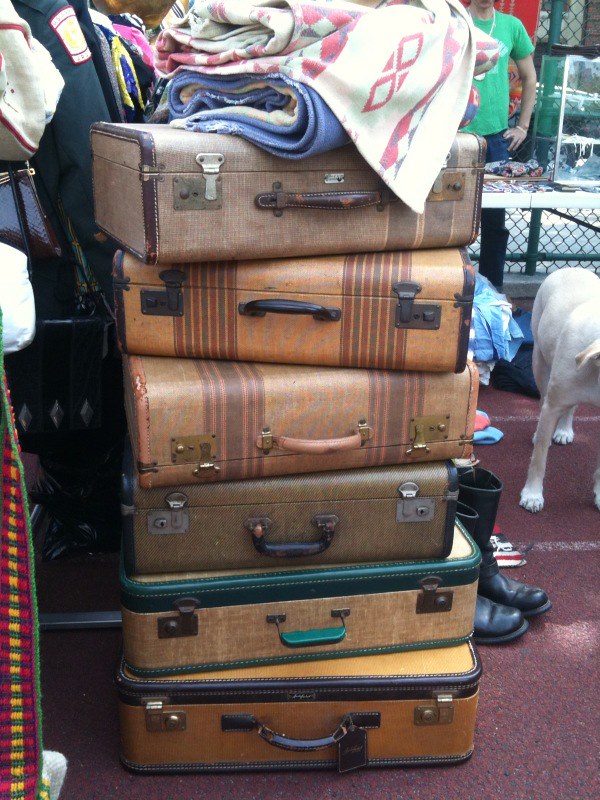In the photo, a bustling outdoor market scene unfolds, resembling a flea market or garage sale. The focus is a stack of six vintage, old-style suitcases, arranged horizontally with their handles and metallic hinges pointing outward. These suitcases have a uniform medium brown color with leather-like reinforcements and vary slightly in shape from curved to rectangular handles. Atop this tower sits a somewhat untidy pile of woven rugs or blankets, featuring designs with colors such as white, pink, and medium periwinkle blue mixed with white. To the right, a white dog, possibly a yellow lab, stands partly visible. A man or boy in a green t-shirt and blue jeans is vaguely seen in the upper right corner, standing behind a table. The lower left corner reveals part of another colorful woven item or belt in red and yellow. Additionally, the toes of a pair of black boots peek into the frame, emphasizing the notion of a sale event. The scene rests on an off-white, off-red, and muted brown outdoor carpet, adding to the eclectic atmosphere of this lively market setting.